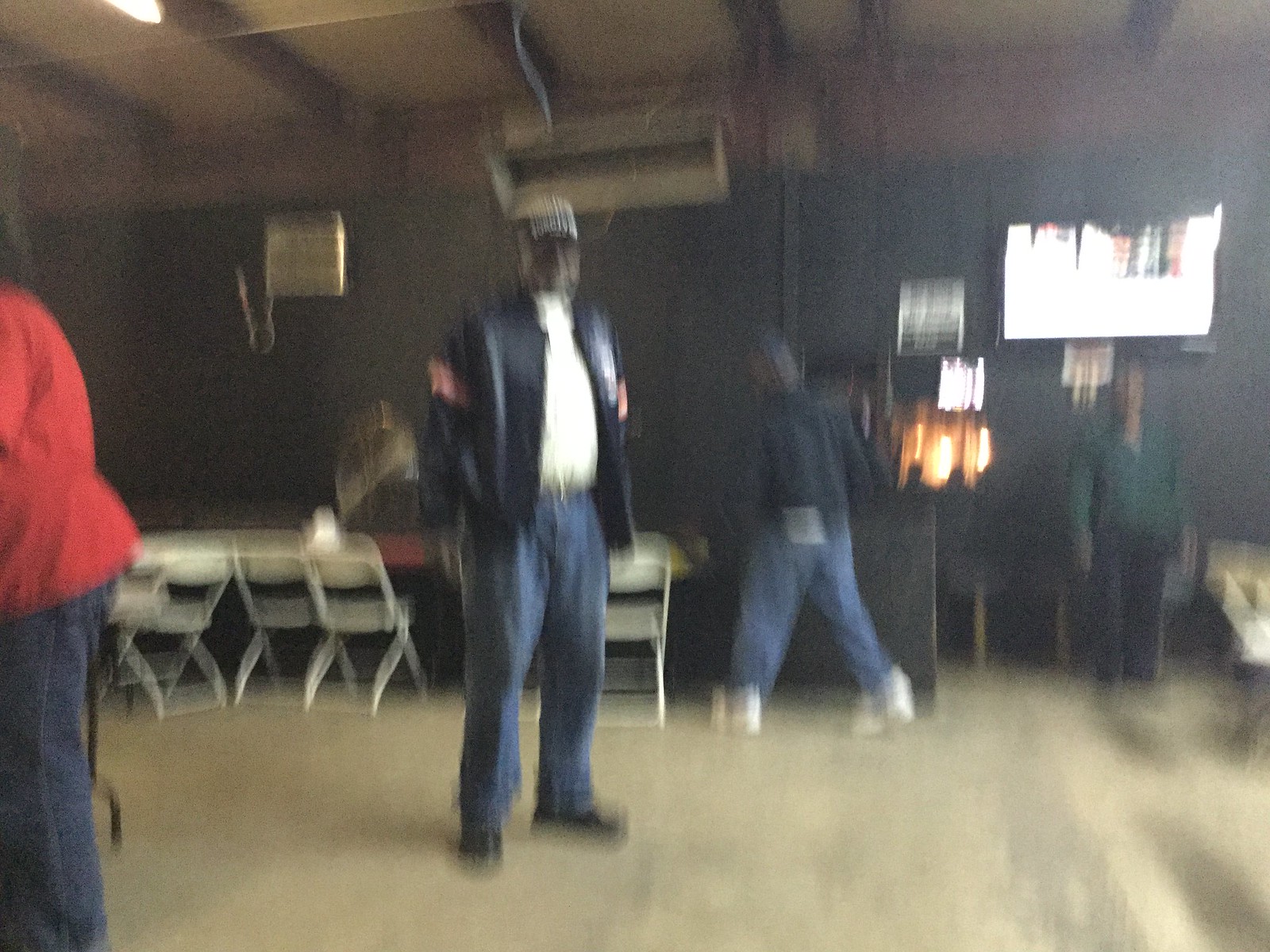In this blurry image, we observe a gathering of individuals seemingly preparing for an event. The focal point is a group of four people situated in a room with dark black walls and a light gray, hard concrete floor. One man, positioned at the center, is notably identifiable with dark black skin, dressed in a black leather jacket with emblems on the upper arms, a white t-shirt, blue denim jeans, a belt, and black shoes, standing and facing the camera. To his right, another person appears clad in a black jacket, blue denim jeans, and white sneakers. Moving further right, a third individual is wearing a green shirt with dark pants. To the far left corner, an additional figure is partially visible, adorned in a red shirt and blue denim jeans. Behind these people, there are several metallic folding chairs arranged next to a long table, illuminated under bright lights. Up on the ceiling, an air conditioning unit can be discerned, and an open window is visible toward the top right of the image. The background walls are painted dark, and exposed brown rafters are prominently visible on the ceiling.